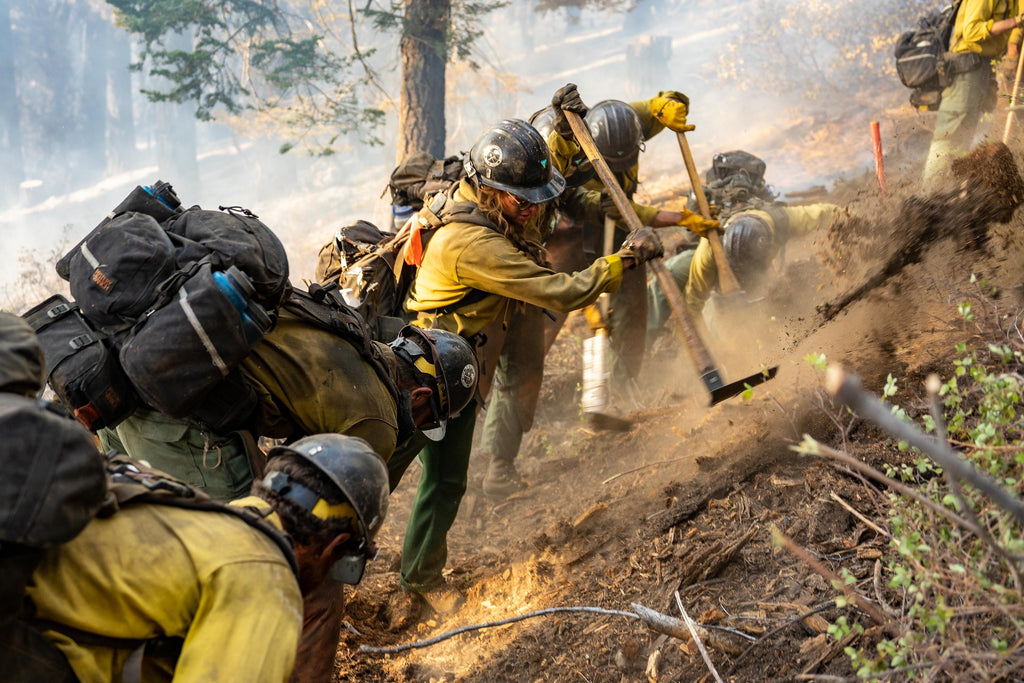In this dynamic outdoor image, a dedicated group of firefighters are fervently working on what appears to be a dig operation amidst a smoky and hazy backdrop of tall, skinny brown trees. These men and women, dressed in yellow jackets, brown or green pants, and black helmets, are energetically digging at the ground, sending mud and dust flying, particularly noticeable on the right-hand side of the image. Some are equipped with tan and black hoes, while others carry backpacks and wear face respirators, emphasizing the intensity and potentially hazardous nature of their task.

The scene is chaotic yet focused, as one can observe a man distinctly holding a blue water bottle amidst the flurry of activity. The ground beneath them is strewn with sticks and leaves, adding to the ruggedness of the terrain they are working on. The bright sunlight filters through, illuminating their determined efforts under the clear, sunny sky. Though their exact mission is unclear, the urgency and seriousness in their movements suggest they might be engaged in rescue operations or clearing debris, tackling the challenges of their environment head-on.